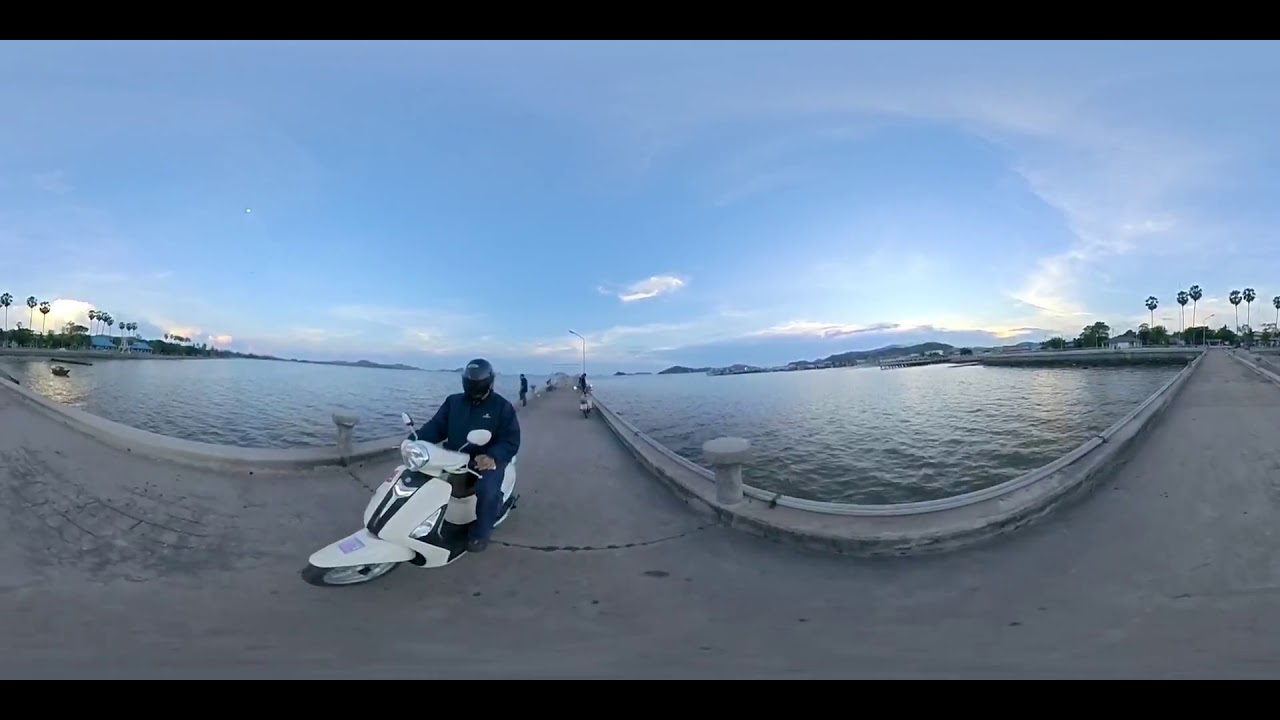The image is a 360-degree fisheye lens shot, offering a wide-angle and slightly skewed perspective. At the center-left of the photograph, a white and black motorbike with wing mirrors and a central light on the handlebars is either parked or moving along a concrete pier. The driver, clad in navy blue protective gear and black shoes, with a dark blue or black helmet and shield down, effectively hides their face. The concrete pier, slightly arched due to the lens distortion, stretches between two calm, cement-bordered reservoir-like bodies of water, framed by distant palm trees on both the left and right sides. Various people dot the edges of the pier, some standing near the water and others positioned along the pathway. The backdrop showcases a lush, tropical environment, with a hilly coastline, palm trees, and even some islands on the horizon. Overhead, the sky is a vast expanse of blue with a few scattered clouds and the sun peeking just above the cloud line.